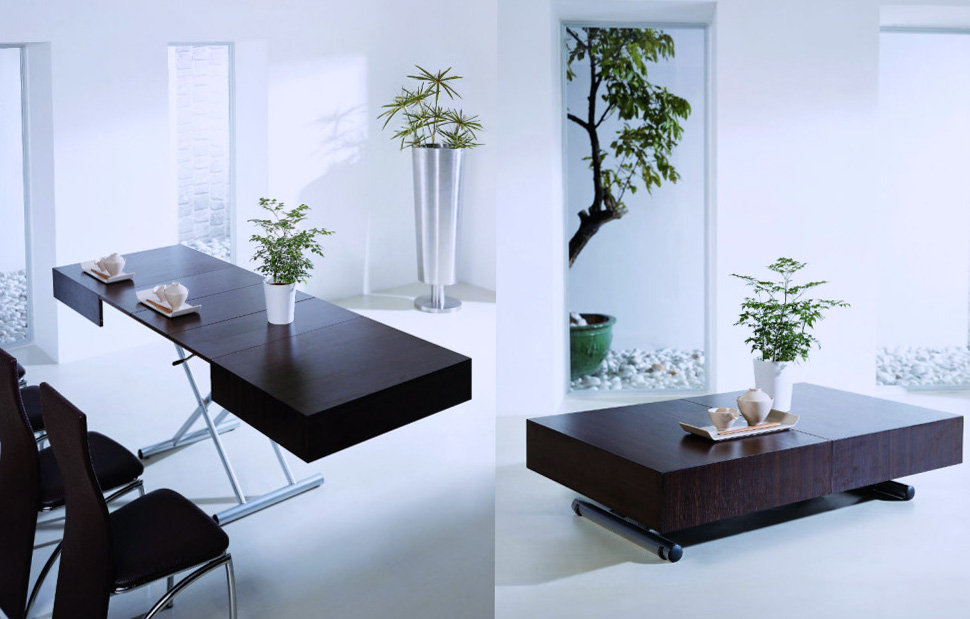In this rectangular image, we see two photographs side-by-side, both depicting a sleek, modern, Asian-inspired living or office space. The left photograph showcases a pristine, all-white room with tall, narrow windows and white floors. Central to the room is a dark, artistically designed desk featuring a steel, ironing board-like stand. A small potted plant sits atop the desk, accompanied by two indistinct objects. At the lower left, three black chairs are neatly lined up. In the corner, a tall, slender silver cylindrical plant holder contains a vibrant plant. The right photograph presents a similar room setup. Here, the desk from the left image has been converted into a low, modern coffee table, maintaining the dark wood finish. This table, like its desk counterpart, holds a small potted plant with a white base. Large rectangular windows reveal a gravel ground outside and a planted tree visible from within, adding a seamless connection to nature. The overall minimalistic, modern aesthetic ties both images together, emphasizing clean lines, simplicity, and a harmonious blend of natural and industrial elements.